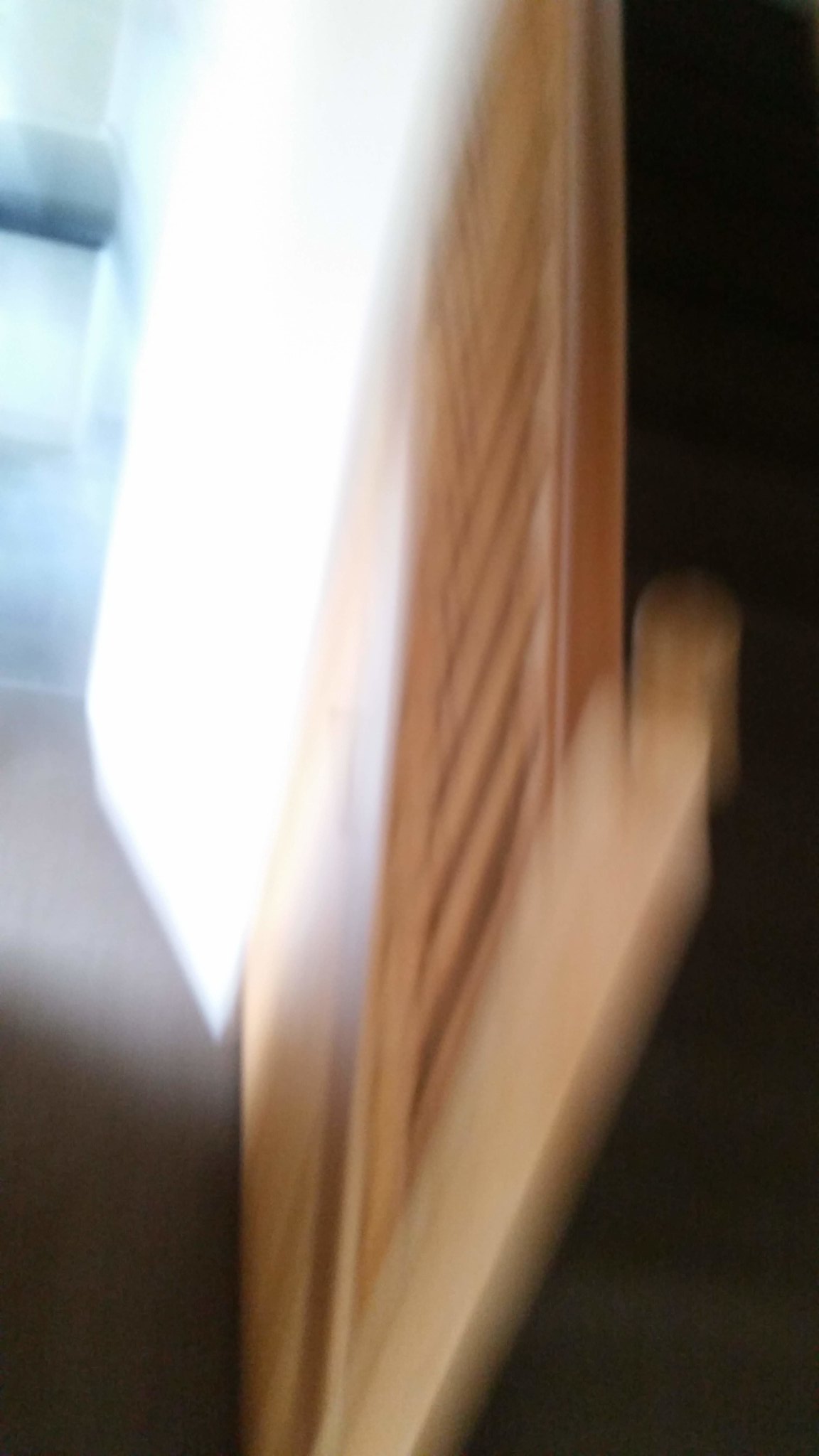This photograph, a tall and narrow rectangle, features an extremely out-of-focus scene. The left-hand side of the image is illuminated with bright white and blue hues, suggesting the presence of a light source, possibly from an open door or window within a building. The right-hand side is enveloped in darkness, devoid of any discernible details. Dominating the middle of the photograph is a wooden structure, characterized by slats and resembling either the banister of a staircase or the headboard of a bed frame. The wood varies in color from light brown to amber and dark brown. Despite the heavy blurring, which makes most details indistinguishable, the central wooden object and the contrast between the bright light on the left and the dark shadow on the right are evident. There are no visible people, animals, plants, buildings, or mechanical objects within this blurred image, emphasizing its abstract and mysterious nature.